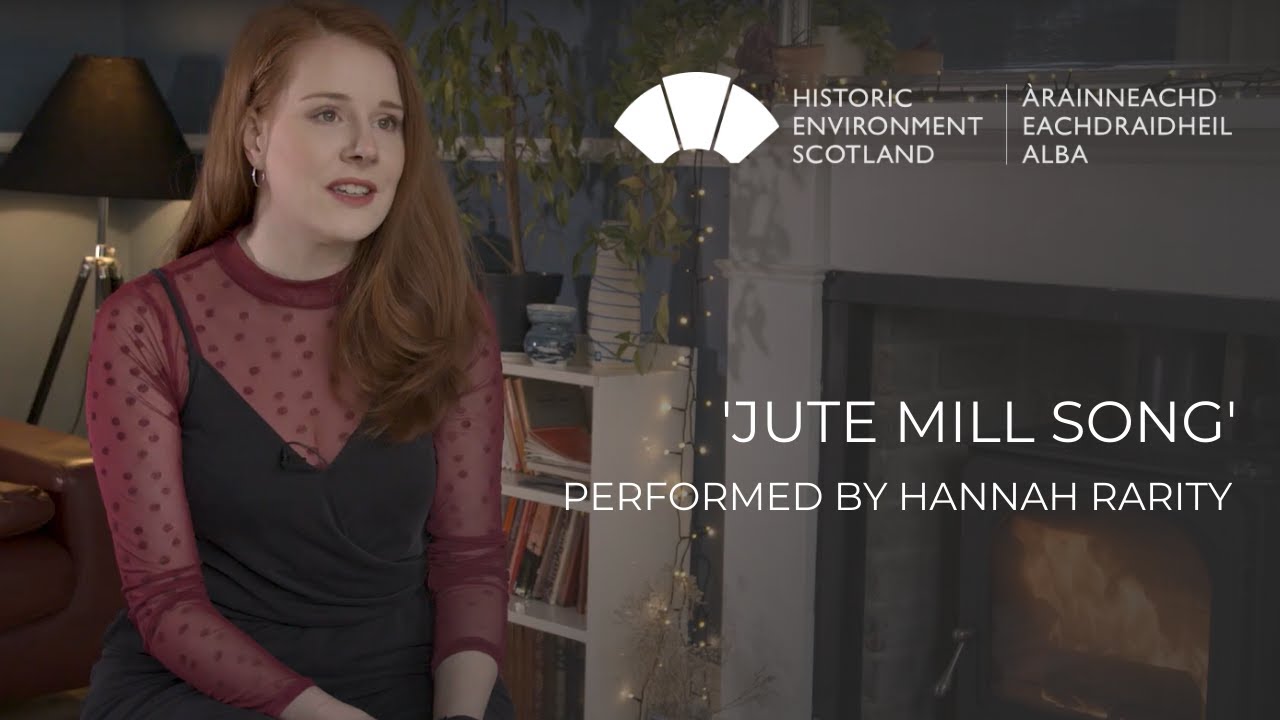In this color photograph, a young woman with reddish blonde, shoulder-length hair sits to the left side of the image, looking slightly to her right with her lips parted in a faint smile. She is dressed in a sheer red top adorned with small hearts and shapes, layered under a black slip dress. She wears earrings and has bluish eyes. Behind her are various room elements including chairs, a lit lamp, and a bookshelf with books and plants. The environment suggests an interview or informal performance setting. To the right of the woman, white text on a dark background reads “Historic Environment Scotland” followed by phrases that appear to be in Gaelic, "Earrainneachd Eachdraidheil Alba," and "Jute Mill Song performed by Hannah Rarity." Centralized is a slightly obscured figure or logo. The background also features a darkened fireplace with a lit fire.